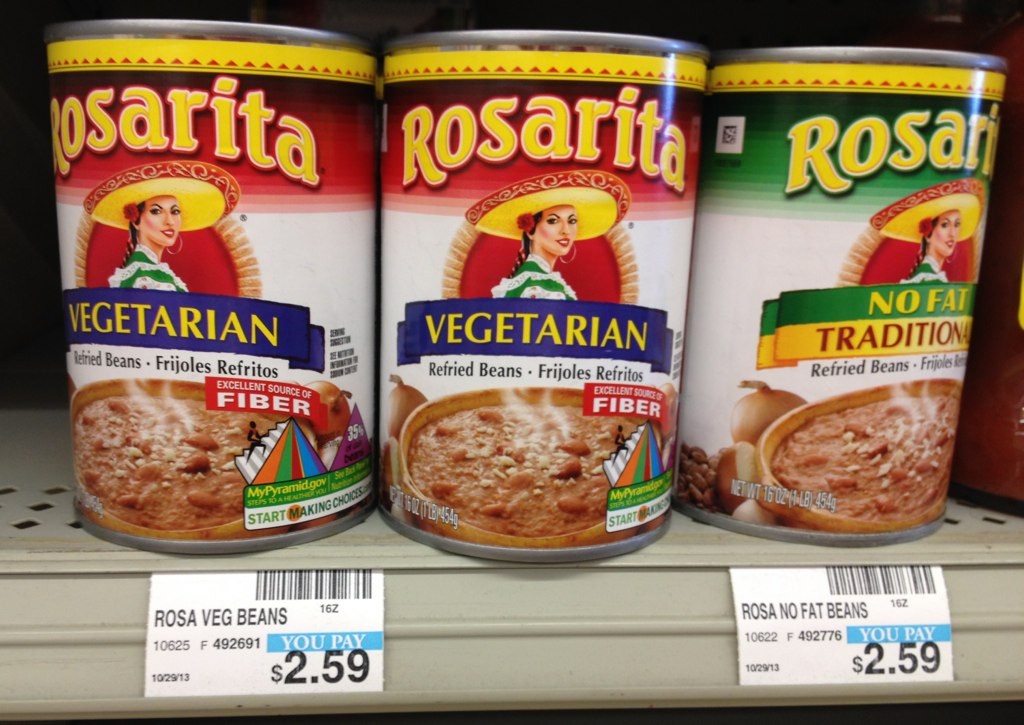Here's a more detailed and cleaned-up caption for the image:

"A close-up view of a grocery shelf displaying three cans of Rosarita refried beans. Each can prominently features the brand's signature image of a Mexican woman dressed in traditional attire with a vivid red sombrero bordered in yellow. 

The left and middle cans are labeled 'Vegetarian', showcasing an appetizing image of refried beans served steaming hot in a wooden bowl. The left and middle cans are priced at $2.59 each. 

On the right is a can of Rosarita 'No Fat Traditional' refried beans, also adorned with the same iconic mascot and priced at $2.59. Despite similar packaging, the left and middle cans cater to a vegetarian diet, while the can on the right offers a traditional no-fat option."